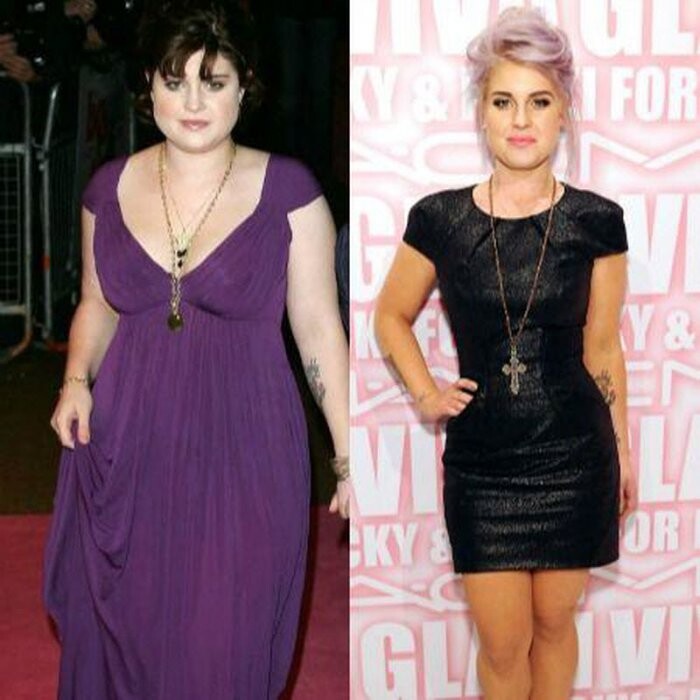This image features a before-and-after comparison of celebrity Kelly Osbourne's weight loss journey, divided into two parts: left and right. On the left side, a younger and significantly heavier Kelly Osbourne stands on a red carpet, dressed in a full-length purple gown adorned with layered gold necklaces. Her dark hair complements the gown, and a distinctive tattoo on her left arm highlights her identity. The right side of the image showcases a transformed, slimmer Kelly Osbourne, now with pink hair, exuding confidence as she stands with her hand on her hip. She wears a chic black mini dress paired with a long necklace featuring a cross. The background displays multiple logos, including MAC, indicating a more recent appearance. This side-by-side presentation underscores her impressive weight loss and style evolution.